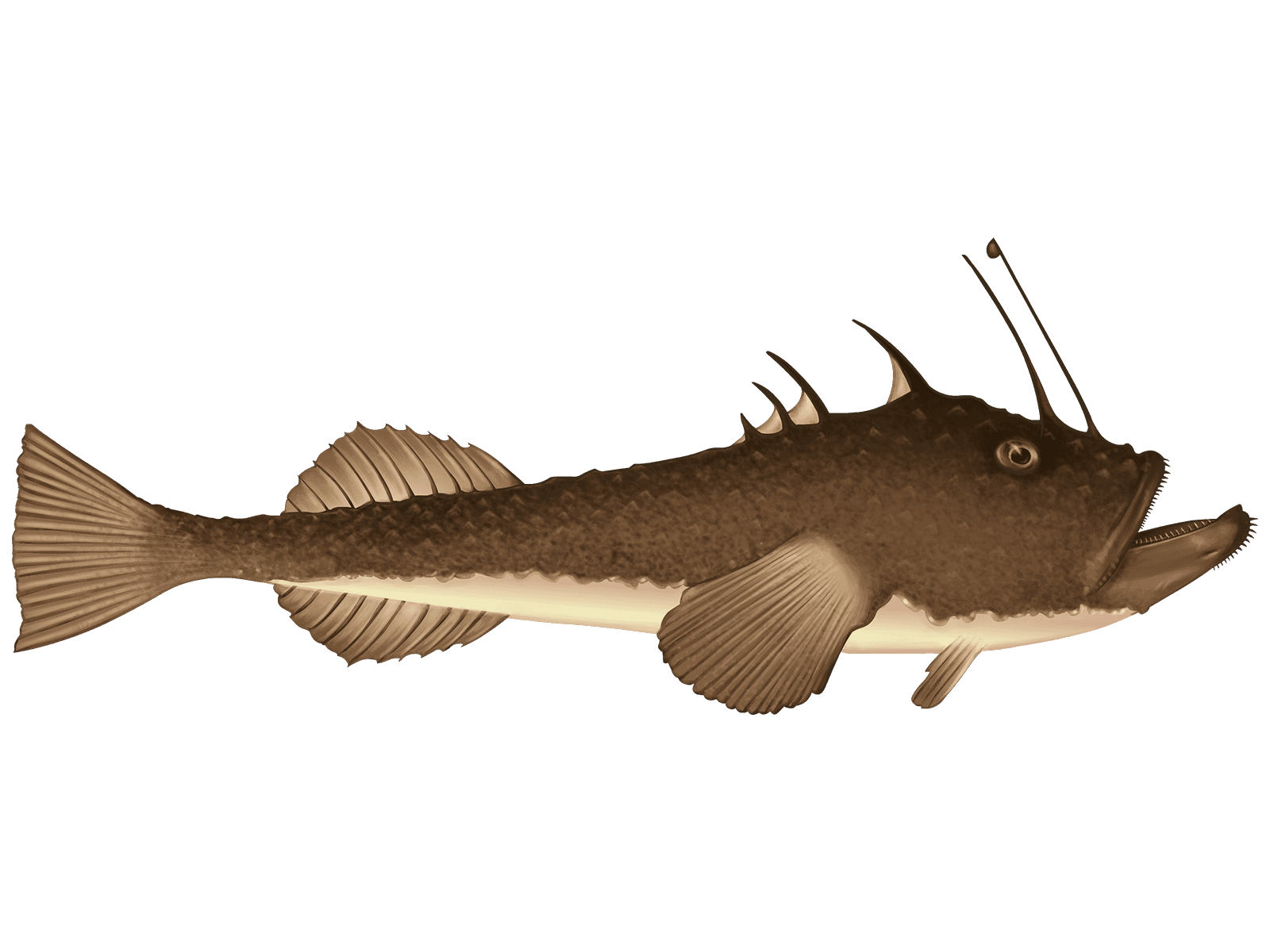This is an illustration of an unknown species of fish, possibly prehistoric or fantastical, displayed against a white background. The fish is oriented with its mouth open, pointing to the right, revealing sharp, small teeth. The lower portion of the mouth appears slightly larger and more pronounced. The body is primarily dark brown with a textured skin, transitioning to a tannish white or cream color on the belly. 

Distinctive features include large, antenna-like bony protrusions or spines on its head—one in front of the eye and one behind, along with an upward-facing mouth with spikes or teeth extending down its chin. A webbing of a tannish color is visible behind these protrusions.

The fins and gills are fan-shaped and brownish, blending elements of dark brown and cream colors. The tail fin is triangular and mermaid-like. Overall, the fish exhibits a mix of anglerfish-like characteristics, particularly the antennae that might resemble those of an anglerfish, although without a visible bioluminescent bulb. The fish's eye is a grayish-brown, contributing to its overall enigmatic appearance, which blends elements of both modern and prehistoric aquatic life.